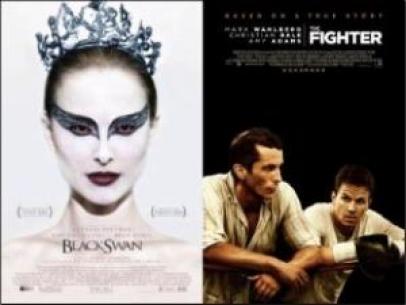Displayed are side-by-side posters for the films *Black Swan* and *The Fighter*. The *Black Swan* poster, on the left, prominently features a close-up of a woman's face, identified as Natalie Portman's character. Her complexion is pasty white, with dramatic, elongated black makeup extending from her eyes outward, giving an intense, almost otherworldly appearance. Her hair is slicked back into a tight bun, crowned with a delicate tiara, suggesting her ballerina role. 

On the right, the poster for *The Fighter* features two men, portrayed by Mark Wahlberg and Christian Bale, leaning against the upper ropes of a boxing ring. Both are dressed in white shirts, with the man on the right wearing boxing gloves. Their poses suggest a moment of introspection or readiness before a match. The film titles are prominently displayed on both posters, though the detailed text is difficult to read. Black Swan's text aligns towards the bottom of the poster, while The Fighter's text is positioned at the top, creating a contrasting visual layout between the two.